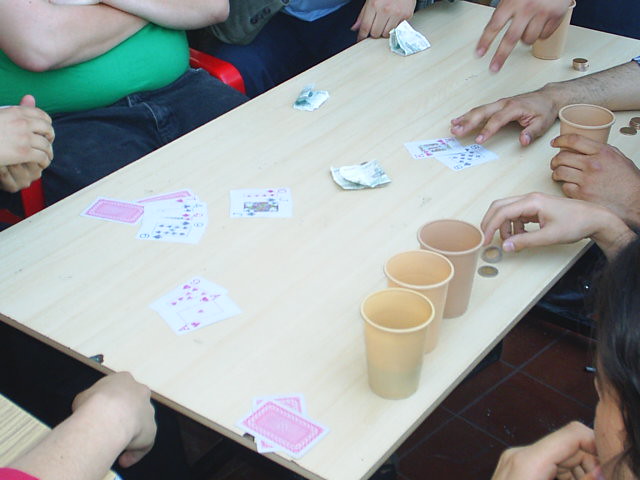The image depicts a lively scene of six people gathered around a light-colored table, deeply engrossed in a game of poker. A variety of items are scattered across the table, including several playing cards, some face up and some face down, along with several bills and coins, hinting at the stakes involved in the game. Positioned around the table are four cream-colored plastic water glasses. 

One of the players, a man in a green t-shirt and jeans, is seated in a red chair with his arms crossed over his chest, showing a bit of a larger belly. Another player's clasped hands rest on the table, though their face remains unseen. There is a partial view of one individual's face, who is wearing glasses and has their hands raised to their mouth, perhaps in contemplation. Another participant appears eager to make a move, with one hand poised to grab a coin on the table.

One player has a firm grip on his plastic water glass with one hand, and the other hand is securing two cards, preparing for the next move. Meanwhile, another participant has his hand stretched out toward the table, likely anticipating his next action in the game. The detailed expressions and varied postures of the players add to the intensity and excitement of the setting.